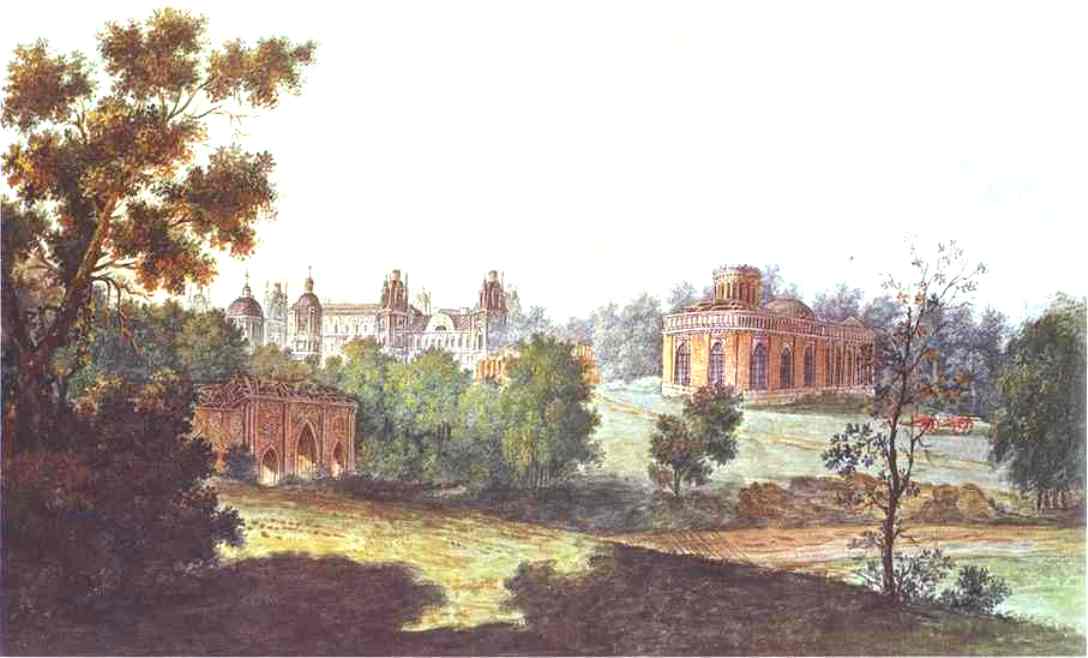The image is an artist's portrayal of a historical rural scene, possibly from the 1800s, featuring a college campus or a similar institutional setting. The scene includes three prominent buildings set within a hilly, green landscape. The largest building on the left has a circular arrangement of columns on its roof, leading to a dome, and is white in color. To its right, but still in the background, another building features three to four domes on its roof and has orange walls. Closer to the foreground, a smaller structure with orange walls is located on the lower left. A notable detail is the shadows cast by trees in the foreground at the bottom of the image. 

The scene includes trees scattered throughout, with a particularly large tree on the left and a smaller one on the right edge. Among the greenery, there is a dirt path connecting the white building to the other structures. The depiction also includes what appears to be an empty wagon or horse and buggy near the right side, partially obscured by a tree. The sky is predominantly white and cloudy, suggesting an overcast day. The main colors used in the painting are green, white, brown, and orange, reflecting the earthy and serene atmosphere of the countryside setting.